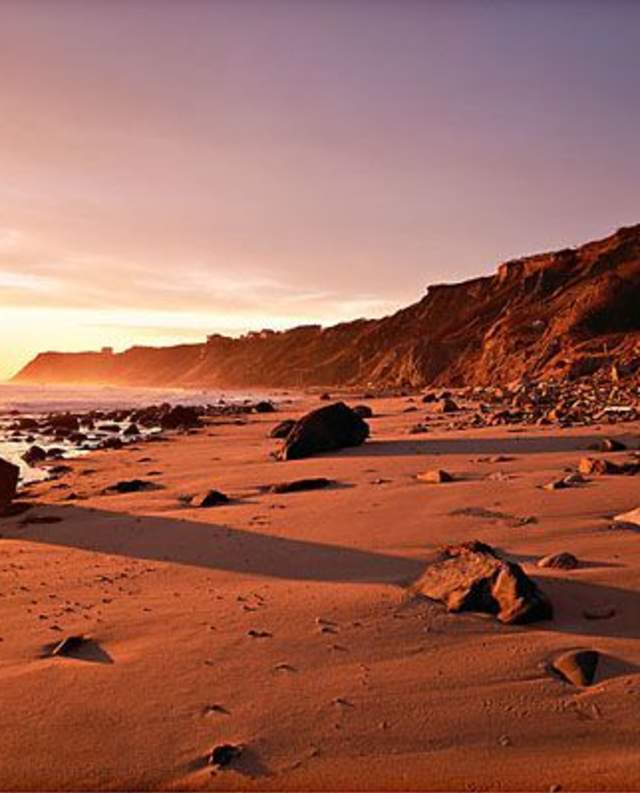This photograph captures a serene sunset scene along a rocky, sandy beach, reminiscent of the California coast, possibly near Malibu. The image features a compacted, clay-colored sandy shoreline dotted with numerous large rocks. Off in the distance to the right, a rugged cliff face or mountain ledge stretches upwards, and some indistinct debris or natural materials can be seen nearby. The ocean is just visible on the left, retreating at what appears to be low tide. The sky is ablaze with hues of purple, pink, and yellow around the horizon as the sun sets, casting long shadows across the beach. The overall atmosphere of the photograph is peaceful and undisturbed, devoid of any people or animals, with the blurry quality of the image adding a dreamlike and tranquil touch to the scene.